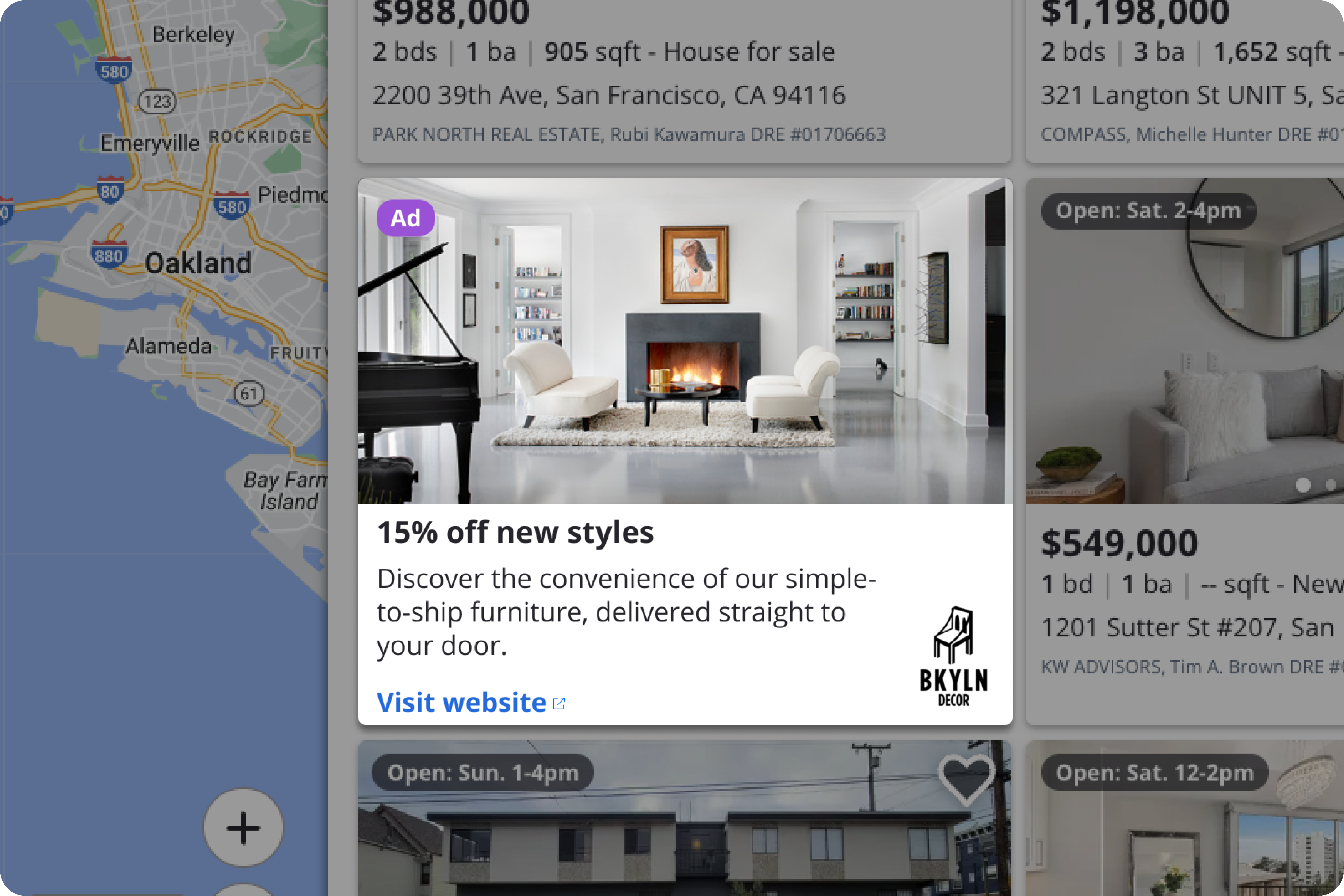A rectangular search box appears over a map, stretching from left to right. The map showcases the San Francisco Bay Area, including locations such as San Francisco, Oakland, Berkeley, and Alameda. Overlaying this map is a highlighted advertisement.

The ad features a cozy living room scene: a lit fireplace surrounded by bookshelves on both sides, with a picture hung above the mantel. In the foreground, to the left, stands an open grand piano. The room also includes two white couches positioned on a white rug atop a grayish floor. 

Below the image, text promotes a 15% discount on new styles, highlighting the ease of shipping furniture directly to your door. A blue "Visit Website" button offers further engagement. The bottom right of the ad bears the logo "BKYLN Decor," featuring a small chair.

Surrounding the ad, multiple listings indicate homes for sale, although they are not the main focus of the image. This detailed scene suggests a robust real estate search activity in the Bay Area.